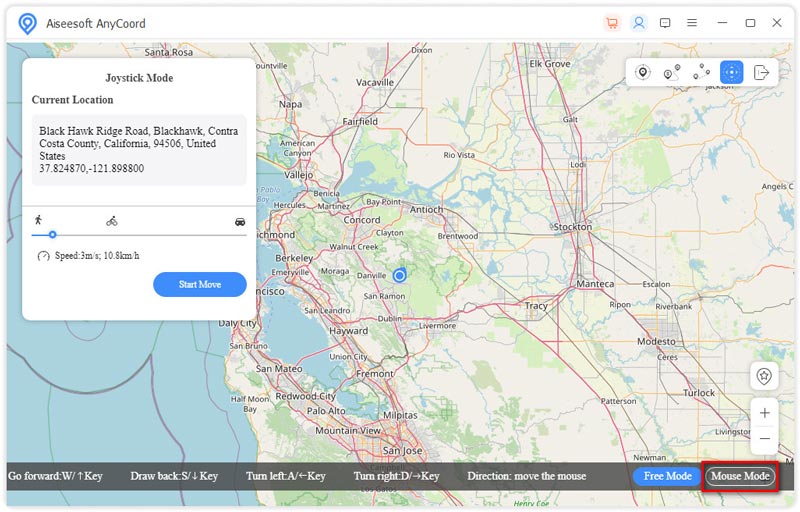The image is a detailed screenshot of a digital map, displaying various notable locations across California. Prominent areas visible on the map include Modesto, Patterson, Fairfield, Napa, Rio Vista, and Palo Alto. In the upper left corner, the text "AICsoft Anycord" is prominently displayed. Below this text, a small box labeled "Joystick Mode" is visible, indicating an interactive feature, alongside the "Current Location," which is detailed as Blackhawk Ridge Road, Blackhawk, Contra Costa County, California, 94506, United States. The precise coordinates provided are 37.824870 latitude and -121.898800 longitude. At the bottom right of the image, there is a noticeable blue button labeled "Start Move."